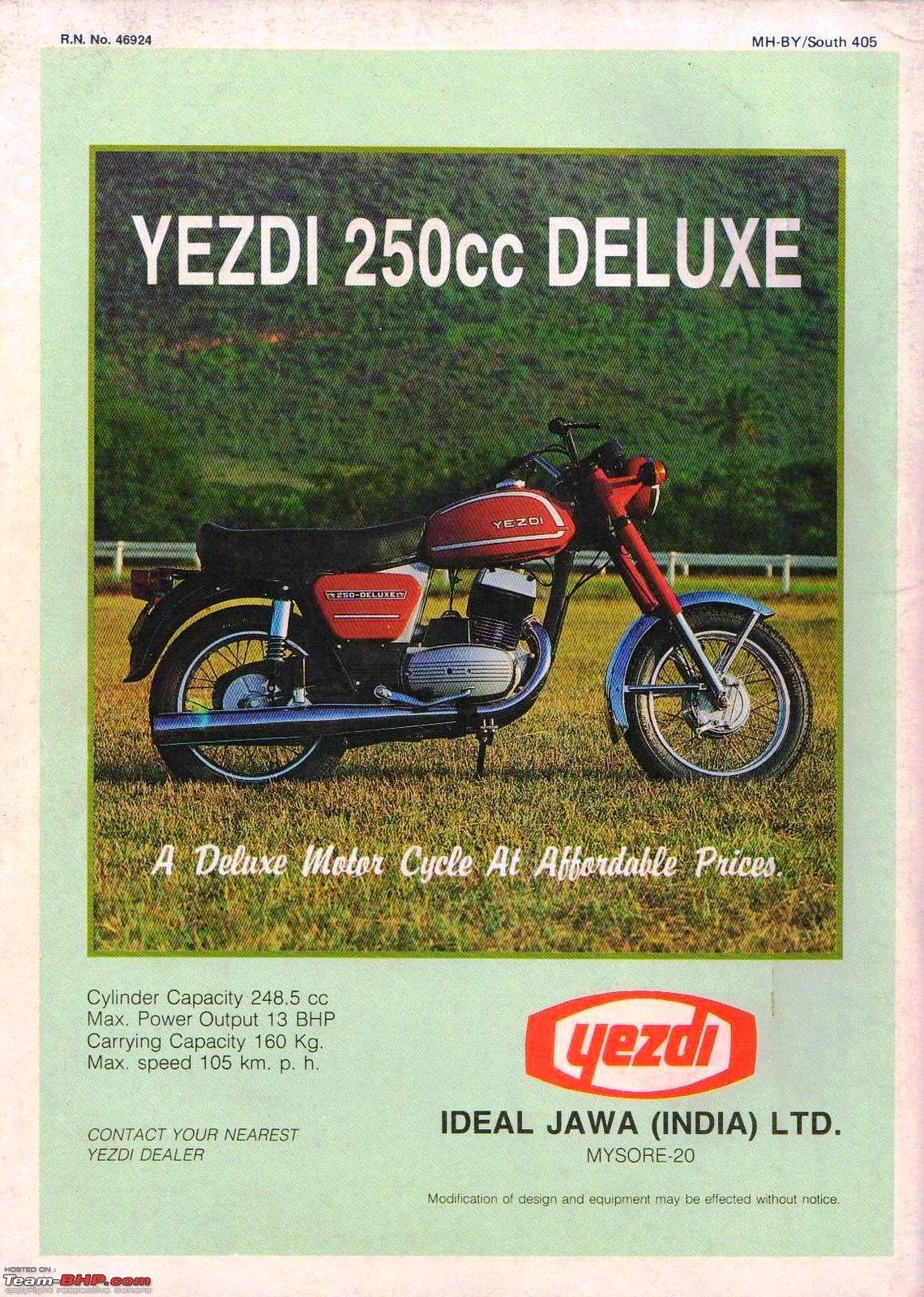The image depicts an old advertisement for a Yezdi 250cc Deluxe motorcycle. The motorcycle, painted red and blue with a polished chrome engine, prominently features "Yezdi" in white letters above the seat. Perched on lush green grass against a backdrop of golden brown and green foliage, the motorcycle appears to be situated at a scenic ranch with a white fence and numerous trees in the distance. The gleaming red fuel tank, adorned with a white stripe and a chrome cap, complements the chrome fender around the front wheel. The bike's handlebar area is black, whereas the arms extending to the front wheel are red. The seating area includes a long, black, rectangular leather seat and a red oil tank underneath. 

Above the motorcycle, in white text, it reads "Yezdi 250cc Deluxe." Below the motorcycle, it says "A deluxe motorcycle at affordable prices" in white text, with additional technical details listed in black text: "Cylinder capacity: 248.5cc, Max power output: 13 BHP, Carrying capacity: 160 kg, Max speed: 105 kmph." The bottom right corner of the image features the Yezdi logo in an oval-shaped design with red edges and white center, accompanied by red text that reads "Yezdi." Below the logo, it states "Ideal Jawa, India Limited, Mysore - 20."